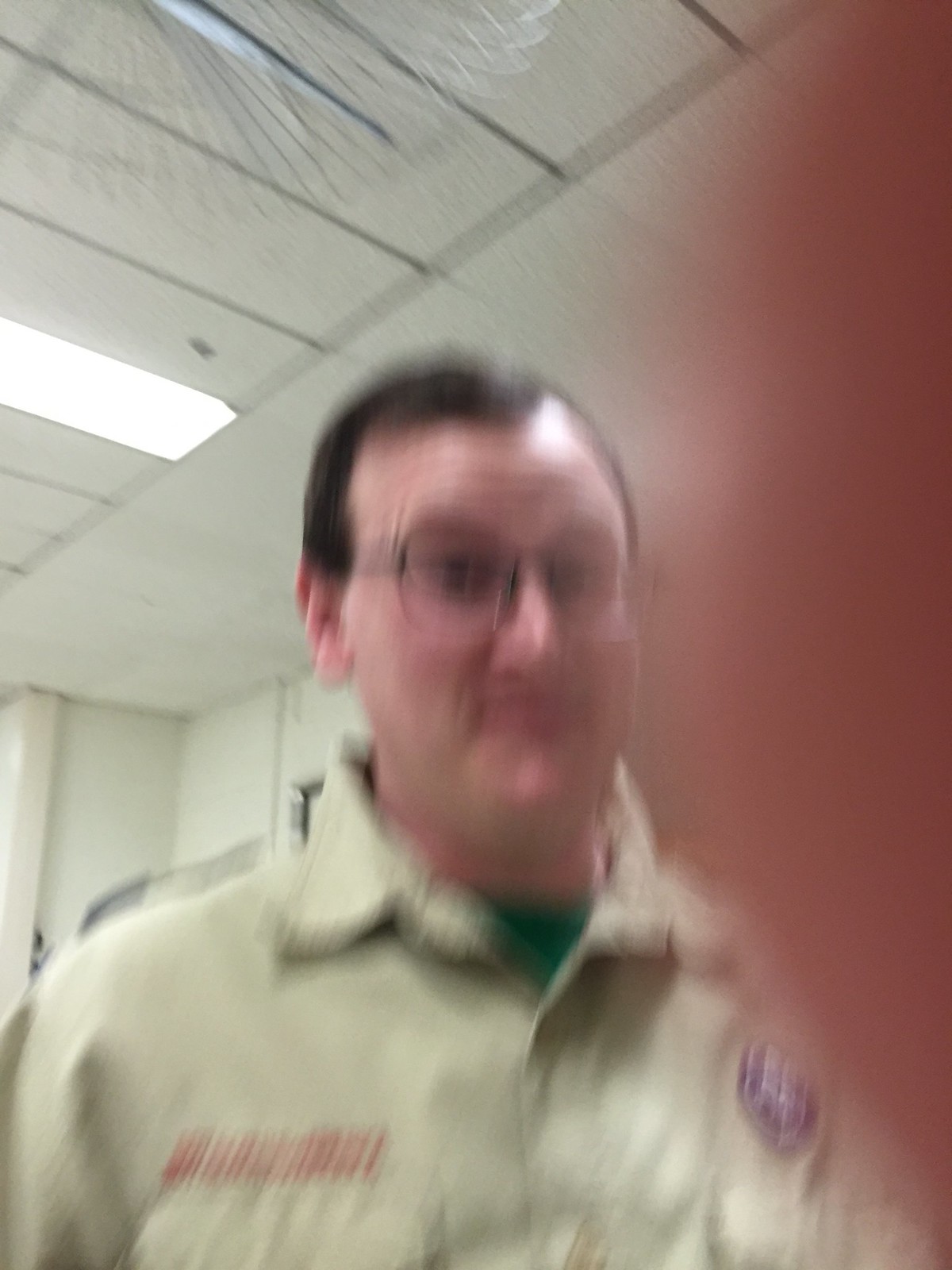This slightly blurry image captures a middle-aged Caucasian man from the chest up. The photographer's finger partially obscures the right side of the picture. Behind the man, a drop ceiling with rectangular tiles and fluorescent lighting is visible. The man's receding hair is short and light or dark brown, and he wears wire-rimmed glasses. He is slightly smiling and dressed in a light tan shirt, adorned with red text above the right pocket and a blue round emblem above the left pocket.